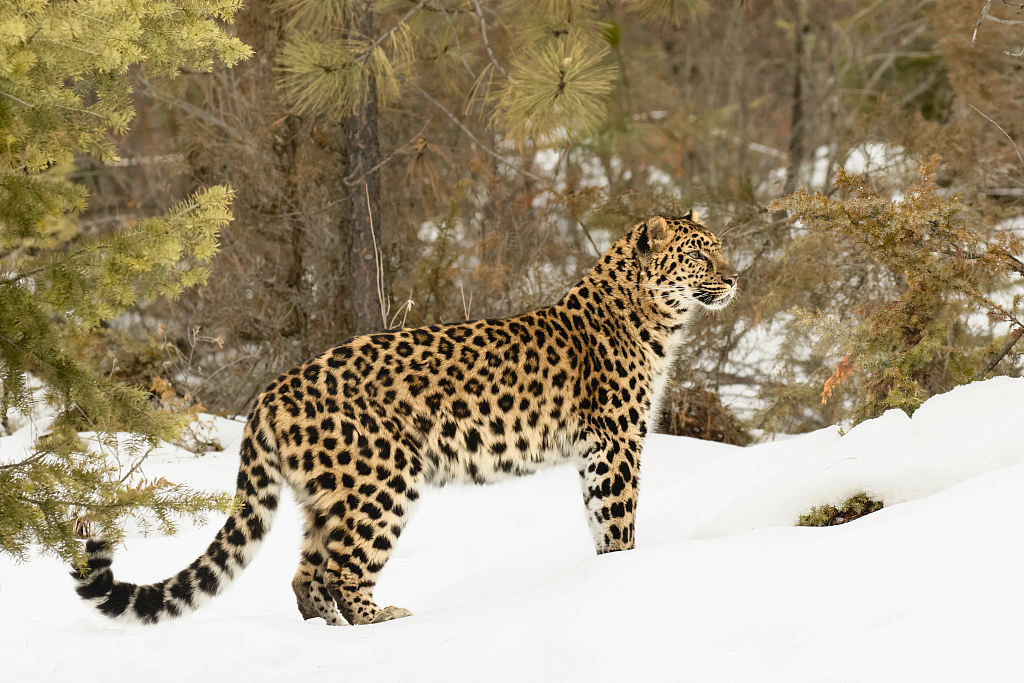In the photo, a majestic leopard stands in a snowy, forested landscape. The snow is deep enough to cover his front paws, reaching over his ankles, while his back paws remain visible. The leopard is intently gazing off to the right, fully focused on something in the distance. His coat is a typical leopard coloration, tan with black and dark tan floret spots, and his white chest contrasts with his spotted belly. His long tail, adorned with similar patterns, curves gracefully. Surrounding him are mostly barren trees, some with sparse brown and green pine needles, including pine trees and one that resembles a Christmas tree in the foreground to the left. The leopard’s serene yet alert posture captures the wild and sparse beauty of the winter scene.